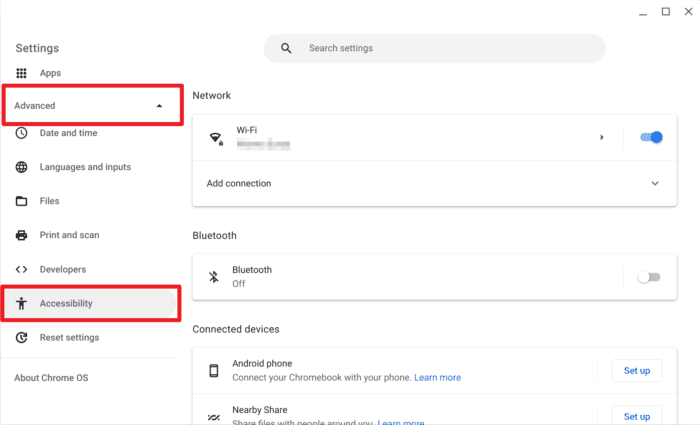The image depicts a webpage titled "Settings" with a prominent search box at the top labeled "Search settings." Various filter options are available, including "Apps" and "Advanced," with the "Advanced" filter highlighted by a red box, indicating it's the focal point for user interaction. Clicking on "Advanced" reveals a dropdown menu with options such as "Date and Time," "Languages and Inputs," "Files," "Print and Scan," "Developers," "Accessibility," "Reset settings," and a section labeled "About Chrome OS."

The "Accessibility" section, also emphasized with a red box, features an icon of a person with outstretched arms, signifying its function for accessing additional relevant settings. 

Further down the page, there is a "Network" section displaying a Wi-Fi status indicator turned on, marked by a blue symbol. An "Add connection" button is also present. Bluetooth functionality is currently turned off, as indicated in the section. The "Connected devices" segment shows an Android phone option with buttons for "Learn more" and "Setup," both in blue. Additionally, the "Nearby Share" feature has a blue "Setup" button, hinting at the capability to share files with nearby individuals.

The entire webpage features a predominantly white background with gray text, providing a clean and clear interface for navigation.